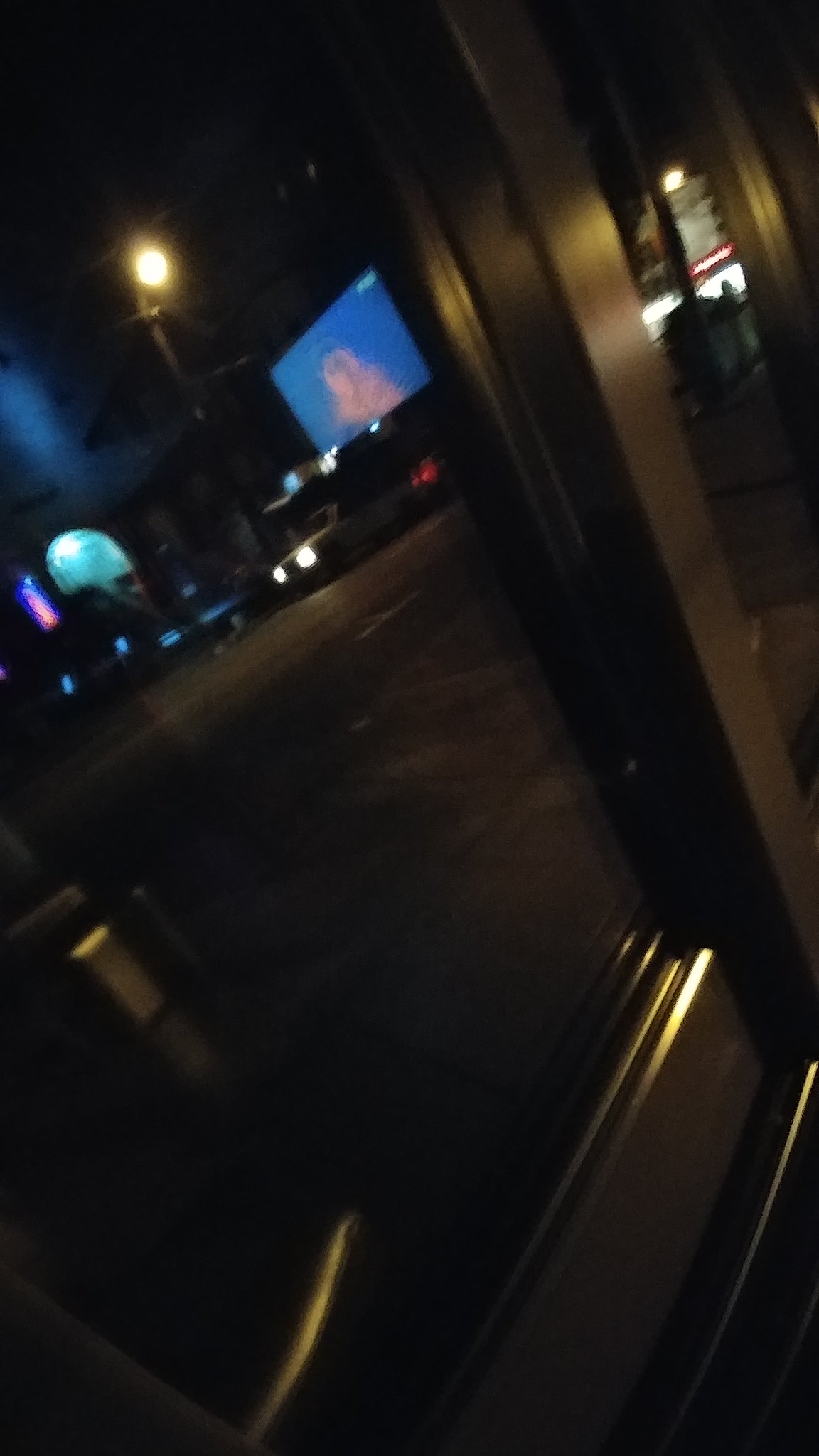The scene is a moody nighttime shot captured from inside a dimly lit restaurant, likely resembling a cozy sit-down diner or a small hamburger joint. The atmosphere outside is decidedly late and dark, with street lights casting a yellowish artificial glow. Through the restaurant's windows, which bear reflections of their own frames and possibly a TV screen or menu from inside, the exterior view reveals a quiet street corner. Directly visible are a few cars, including a truck with its headlights on, parked on the neighboring road. A significant streetlight throws light onto the street where the truck is parked. Across the way, a second building with a prominent bluish-lit window and possibly a purple neon sign stands out amidst the darkness. The visual details suggest an urban setting with a calm nighttime ambiance, punctuated by reflections and glowing screens.